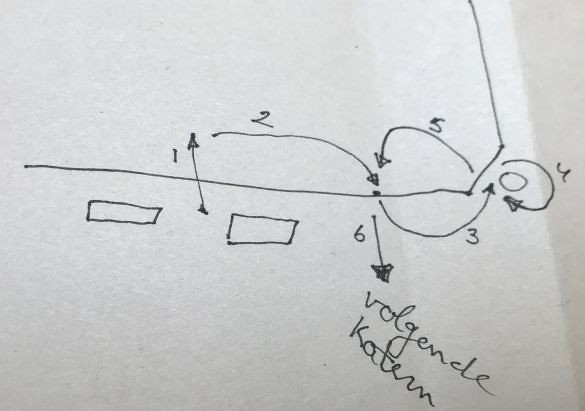**Detailed Schematic Drawing Caption:**

The image is a photograph showcasing a detailed hand-drawn schematic on a white piece of paper. Central to the schematic is a horizontal line that runs directly across the middle of the paper. Approximately at the three-fourths mark from the left, an angled line extends upward at a 60-degree angle for about an inch, after which it proceeds vertically to the top edge of the paper.

Below this horizontal line, there are two small squares spaced about an inch apart. Between these squares, an arrow pierces through the central horizontal line, labeled with the number '1'. Another arrow extends from this '1' arrow, bends, and points to a different location on the central horizontal line, marked as '2'.

From the point where the angled line starts, another arrow originates from the middle of this slant and points to the '2' arrow. Additionally, a third arrow commences from the same point on the opposite (lower) side of the horizontal line and points downward, labeled with the number '6'. The '6' arrow is positioned south of the central line, while the initial two arrows are north.

Remaining below the central horizontal line, another arrow curves from the same originating point and aims at the slanted one-inch line, signed as '3'. Yet another arrow forms a circular motion around the central line. The interior of this circular arrow contains a zero, while its exterior bears the number '4'.

At the bottom of the paper, the phrase "Volgenby Keturn, Keturn" is written in a slanted fashion.